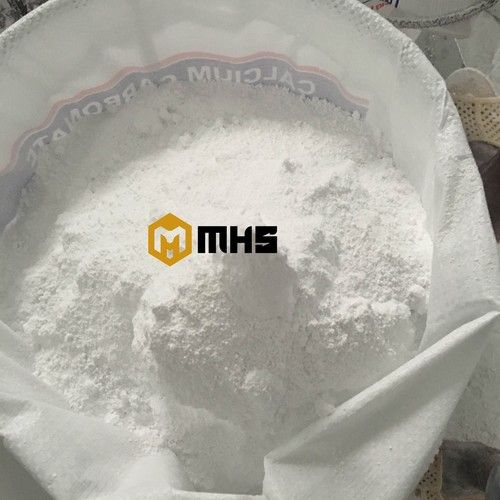The image features a white bag filled with a bright, fine white powder, identified as calcium carbonate. The bag, resembling a garbage can with a circular opening, shows both an outer and inner perspective of its contents. The lettering "calcium carbonate" appears mirrored on the bag, written in white on a blue rectangle with a red stripe at the top. Centered and slightly left in the image, a watermark displaying "MHS" in black and a yellow hexagon with a cut-out letter "M" overlay the scene. The setting includes various items scattered on the ground, such as a pair of white sandals, hinting at an indoor location, possibly a shop. The color palette includes white, tan, brown, black, yellow, and red.